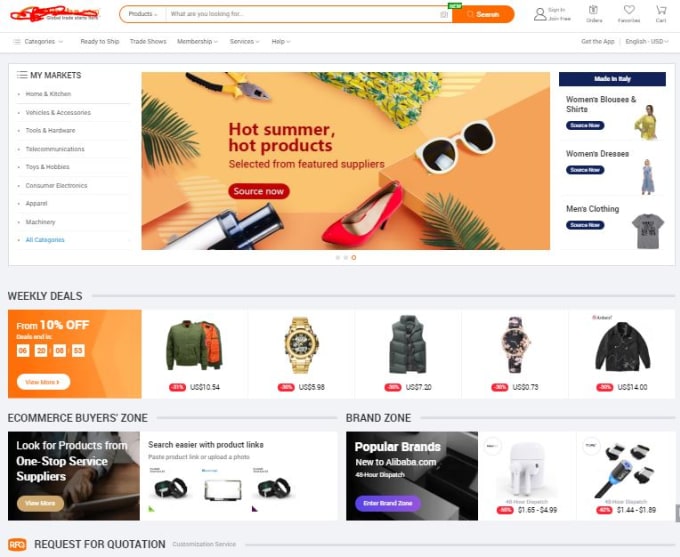This detailed screenshot captures a vibrant online shopping website, which might be Alibaba or a similar marketplace, although the top branding is blurred. Dominating the top of the page is a search bar for product queries. Beneath this, a prominent banner showcases "Hot Summer Products," displaying visuals of items such as sunglasses, shoes, and a hair dryer, urging users to "Source Now" to resell these items on platforms like Amazon.

The left-hand side of the page features a menu labeled "My Markets" with categories including "Home and Kitchen," "Vehicles and Accessories," "Tools and Hardware," and more, indicating a diverse product range available for various market needs. To the right of the banner, specific categories are highlighted, such as "Women's Blouses and Shirts," "Women's Dresses," and "Men's Clothing," each accompanied by corresponding images for easy navigation.

Below the central banner, sections for weekly deals prominently advertise discounts on items such as jackets, watches, and other apparel. The "Ecommerce Buyer Zone" offers streamlined options for sourcing products from one-stop service suppliers, enhancing search efficiency with direct product links. Additionally, the "Brand Zone" spotlights popular brands with quick dispatch options, showcasing electronics like headphones and chargers for quick access.

Overall, the website's layout is user-friendly and meticulously organized into various product categories and promotional sections to optimize the shopping experience. At the bottom, there's a "Request for Quote" feature, suggesting that bulk purchasing is a key component of this marketplace, catering to those looking to buy in large quantities.